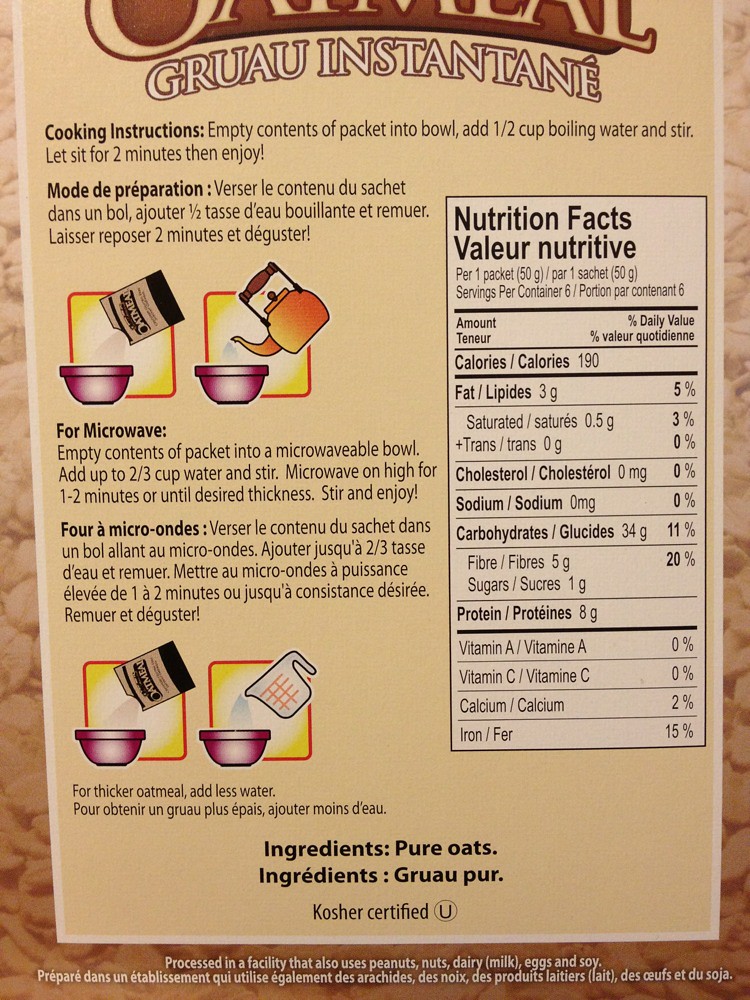This image captures an extreme close-up of the backside of an oatmeal box, placed on a wooden table. The box is bordered in brown, complemented by a white or tan line that frames a beige background. At the top, the word "Oatmeal" is prominently displayed in curved letters with either black or brown shadowing, though partially cropped. Below, it reads "GRUAU Instantané" in a foreign language, likely French.

The box provides detailed cooking instructions in both English and French. The instructions are visually supported by graphics illustrating the process: pouring oatmeal from a packet into a bowl, adding hot water with a tea kettle for stovetop preparation, and using a measuring cup of water for microwave instructions to achieve a thicker consistency. 

The right side of the box features the nutrition facts in a white box with black lettering, detailing that each packet of oatmeal contains 190 calories, 3 grams of fat (5% daily value), no cholesterol or sodium, 34 grams of carbohydrates (11% daily value), 5 grams of fiber (20% daily value), and 8 grams of protein. It also notes the micronutrients, indicating no Vitamin A or C, 2% daily value of calcium, and 15% daily value of iron. Underneath all the instructions, it mentions the ingredients as pure oats and kosher certification.